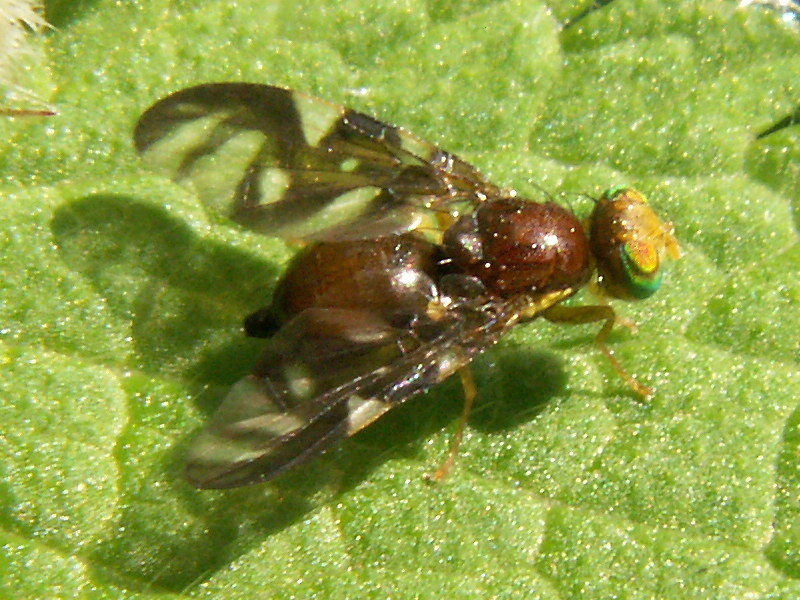This image is an extreme close-up of a fly resting on a glimmering green leaf. The leaf itself appears almost shimmery, with flecks of gold reflecting off its surface. The fly is detailed prominently, with its bright orange eyes and an aquamarine-green face. The fly's body, a rich coffee brown, features distinctly patterned wings that are alternately brownish-black and clear. Its legs, which are yellowish-green, are positioned with two in the forefront and two on the opposite side, adding to the intricate sight of the insect. The fly is just resting there, without any other flies or food around. The overall scene captures the fly's detailed anatomy and the shimmering surface of the leaf, creating a striking and vivid image of this common insect in a moment of stillness.